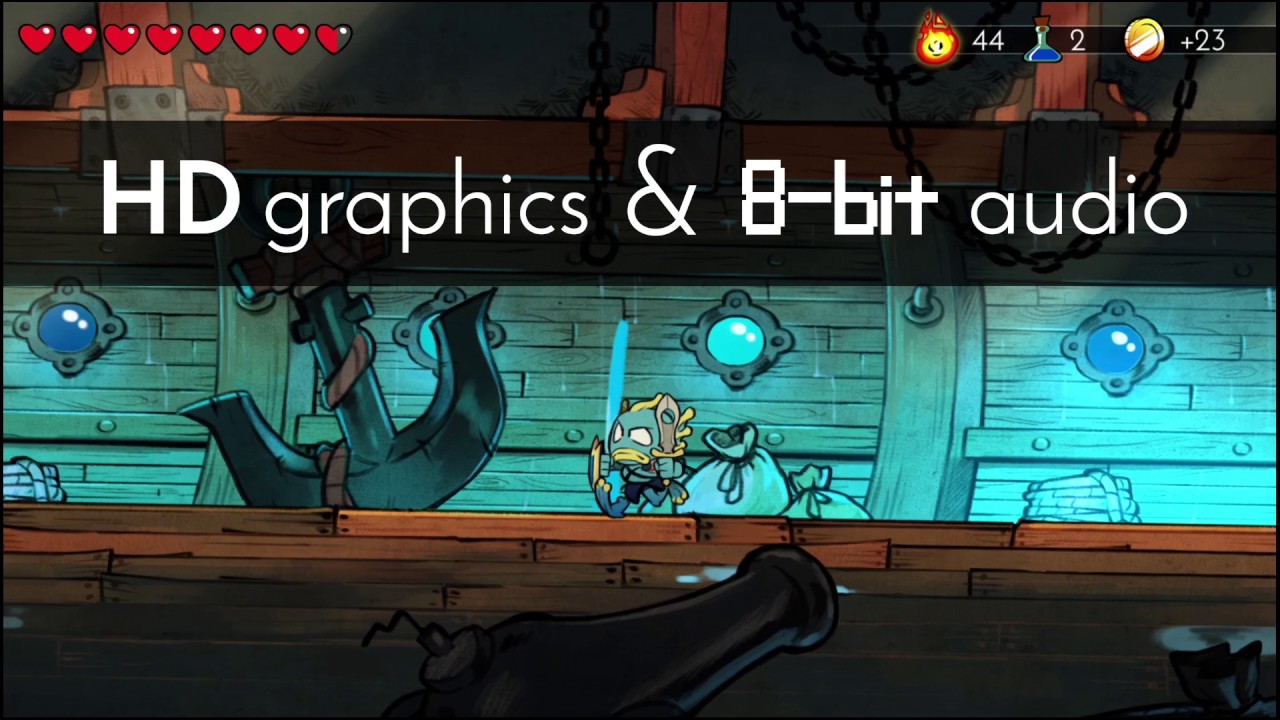The image is a vibrant, cartoon-like scene resembling a screenshot from a video game. Centered in the image is a dark charcoal gray anchor surrounded by an array of detailed elements. Near the anchor, there is an angry cartoon fish alongside some bags. At the top left corner, a series of eight red hearts line up, indicating a health or life meter. On the top right corner, three distinct icons are displayed: a burning yellow smiley face with the number 44 next to it, a beaker with the number 2, and a reddish-yellow disc shape with a plus 23 notation. The text "HD graphics" and "8-bit audio" appears prominently on the image, with "HD graphics" in a clean sans-serif font and "8-bit" in a pixelated font, highlighting the visual contrast between modern and retro elements in the design.